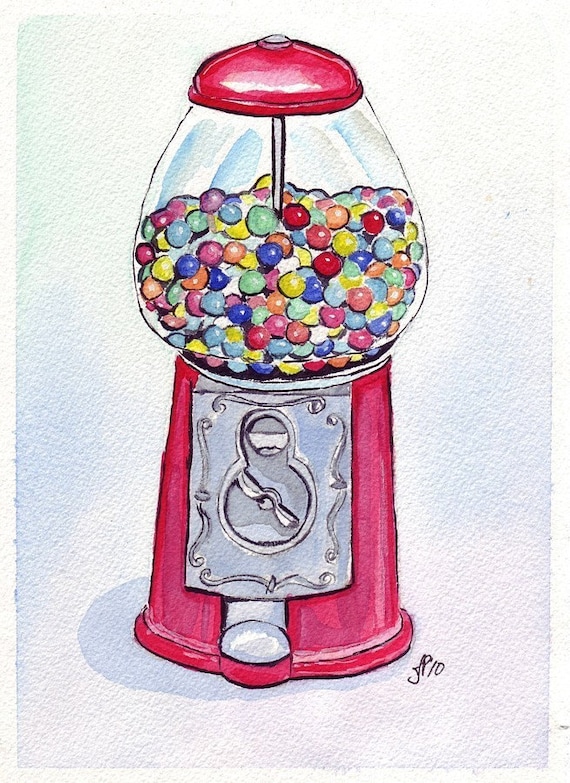This watercolor painting vividly depicts an old-style gumball machine with a glass container at the top, filled about halfway with an array of colorful gumballs. The gumballs are rendered in a spectrum of colors including red, yellow, blue, green, white, orange, pink, and purple, creating a vibrant and cheerful visual. The gumball machine itself is predominantly red, featuring a metallic lid at the top and a silver frontal plate with an ornate pattern. This plate houses a coin slot and a twisting mechanism to release the gumballs. The background of the painting is a soft, light shade of sky blue, providing a subtle contrast that makes the gumball machine and its contents stand out effectively. Overall, the painting captures the nostalgic charm of the classic candy dispenser with intricate details and a delightful color palette.